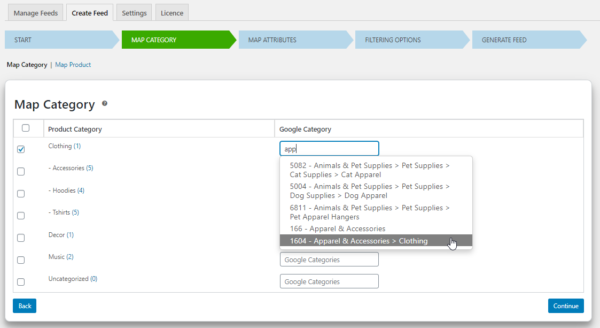This is a screenshot of a web page's interface showcasing the "Create Feed" section, indicated by a clicked tab at the top of the screen. Users also have the option to navigate to other sections titled "Settings" and "License," but the current focus is on "Create Feed." At the top of this section is a sequence of arrows, each indicating a step in the feed creation process. The sequence starts with a blue arrow labelled "Start" on the left, followed by a green arrow labelled "Map Category" to its right, which then leads to a blue arrow labelled "Map Attributes." This is followed by another blue arrow labelled "Filtering Options," culminating in the last arrow on the far right labelled "Generate Feed."

Beneath this sequence is the "Map Category" section, which is selected, displaying various categories on the left side of the screen. Each category is accompanied by a white box with a gray outline that can be clicked. The selected category is "Clothing" (denoted by a number 1 in parentheses), indicating one subcategory or item within it. Other categories listed include "Accessories" (5), "Hoodies" (4), "T-Shirts" (5), "Decor" (1), "Music" (2), and "Uncategorized" (0).